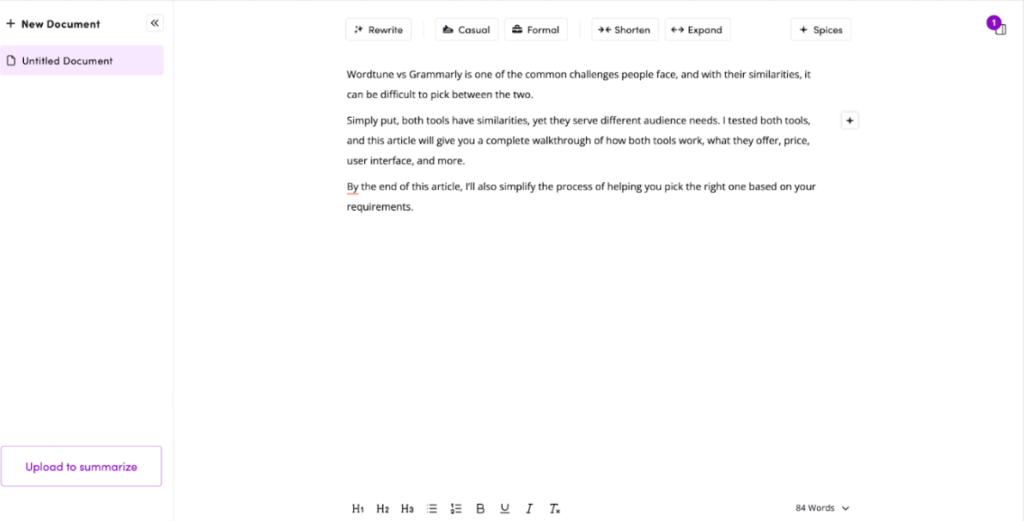The image showcases a screenshot of a digital document editing interface. At the top, the title reads "New Document," followed by a subheading stating "Untitled Document." The interface features various editing buttons, including options for "Rewrite," "Casual," "Formal," "Shorten," and "Expand." Additionally, there's a "Spices" category, likely for adjusting the tone of the text. A shopping cart icon with a purple circle displaying the number one is also visible, suggesting an item in the cart.

The document's text discusses the comparison between WordTune and Grammarly, noting that choosing between the two can be challenging due to their similarities. The author mentions that both tools cater to different audience needs and that the article will provide a detailed walkthrough of their functionalities, offerings, pricing, user interfaces, and more. The aim is to help readers decide which tool best suits their requirements by the article's conclusion.

At the bottom of the interface, typical word processing tools for formatting the text, such as bold and italic options, are available. The document comprises 84 words in total. The background is predominantly white, while the text and various buttons are in shades of black.